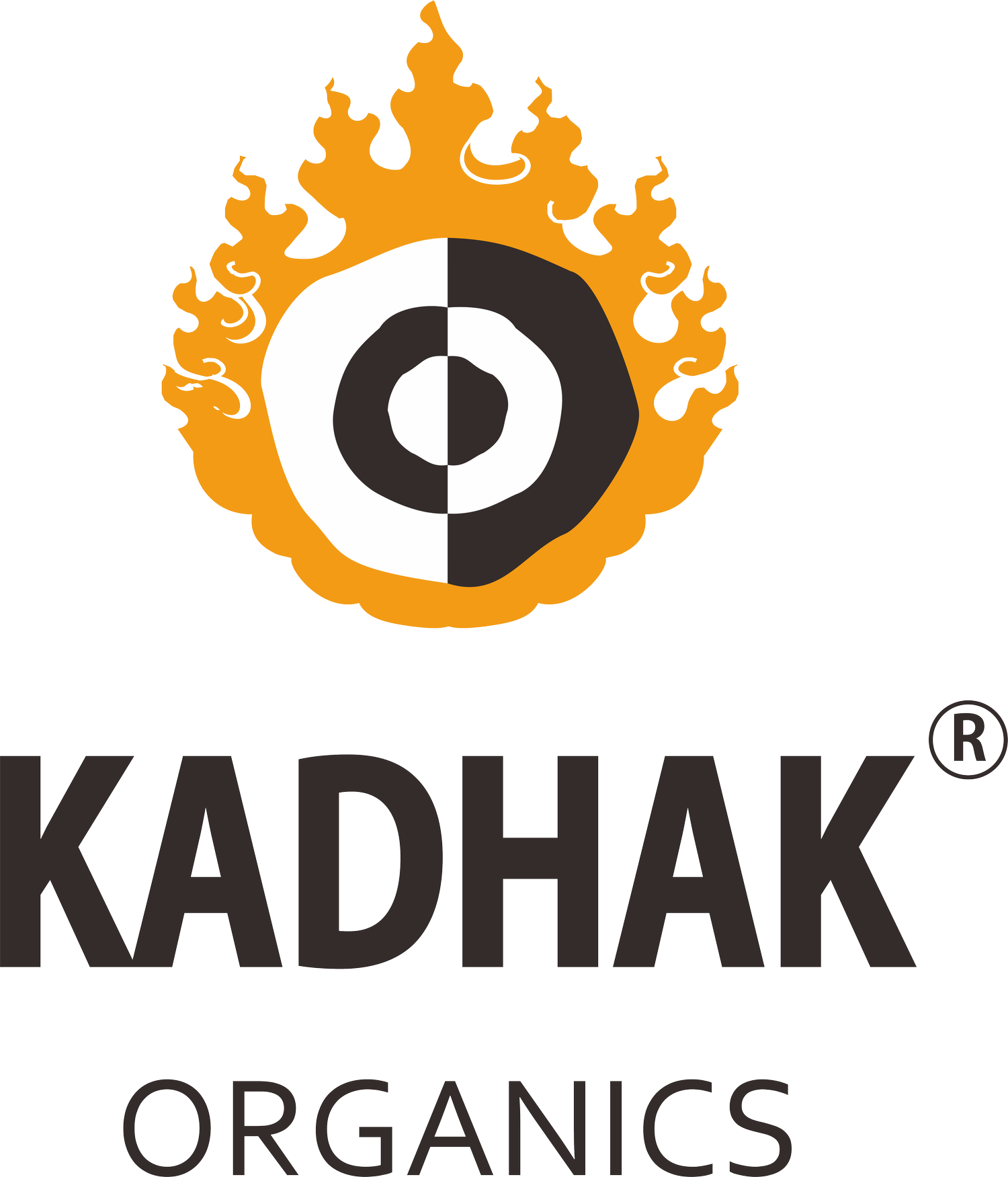The image features a logo set against a white background. At the top, an orange flame-like design encircles a series of three concentric circles. Each concentric circle is split in half vertically with alternating black and white halves: the outermost circle has a left half in black and a right half in white; the middle circle has a left half in white and a right half in black; and the innermost circle mirrors the outer circle with a left half in black and a right half in white. The contrasting colors of the circles create a target-like appearance, but the divisions do not align perfectly. Below this emblem, in large, bold, black capital letters, it reads "KADHAK", accompanied by a registered trademark symbol (®) above the last 'K'. Underneath, in smaller, gray capital letters, it says "ORGANIX".